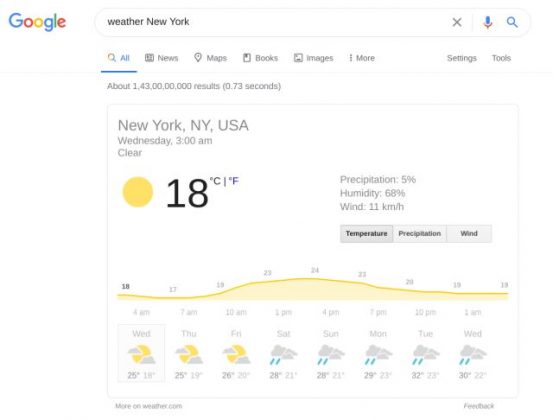The image captures a computer screen displaying a Google search page for the weather in New York, New York, USA. The background of the page is entirely white, and the top search bar contains the query "weather for New York." Below the search bar, there are various options: "All," "News," "Maps," "Books," "Images," and "More." To the right of these options, the strip includes settings for "Settings" and "Tools," and it mentions approximately 1.43 million results were found in 0.73 seconds.

The weather information for New York is prominently displayed, indicating that at 3 a.m. on Wednesday, the temperature was 18 degrees Celsius, with an option to convert to Fahrenheit. Additional weather details are provided, including 5% precipitation, 68% humidity, and a wind speed of 11 kilometers per hour. The page also features a weekly weather forecast visualized by a yellow line representing temperature variations. Each day's forecast includes icons depicting conditions like sunny or rainy, accompanied by high and low temperature estimates.